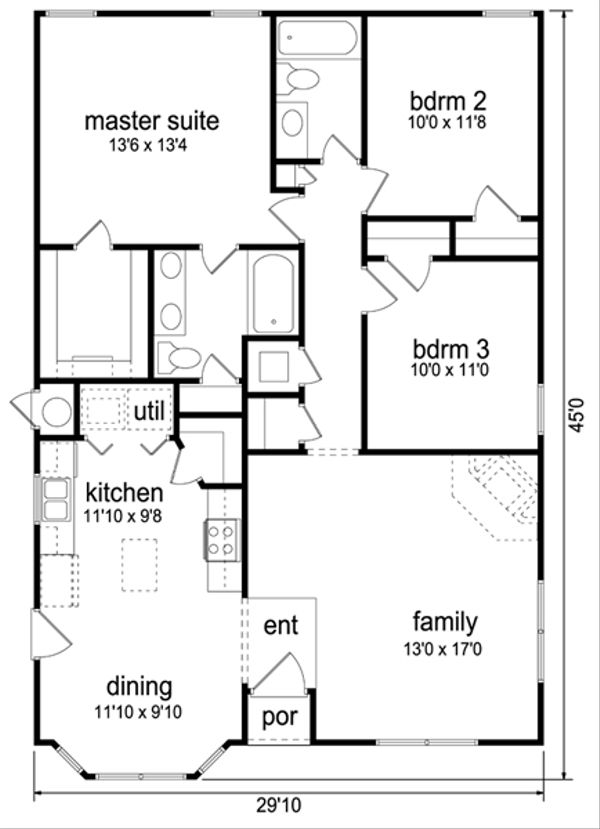This detailed layout plan depicts a one-story house with dimensions of 29 feet 10 inches by 45 feet. In the top left corner, the master suite measures 13 feet 6 inches by 13 feet 4 inches. Adjoining the master suite is a walk-in closet and an en suite bathroom equipped with a double sink, toilet, and bathtub area.

To the right of the master suite lies Bedroom 2, which measures 10 feet by 11 feet 8 inches. A hallway runs between the master suite and Bedroom 2, leading to an additional bathroom. Below Bedroom 2, Bedroom 3 is positioned, measuring 10 feet by 11 feet.

In the bottom right corner, there is a spacious family room measuring 13 feet by 17 feet, featuring an area designated for a fireplace at the top right. Moving left from the family room and beneath the master suite's walk-in closet, is the utility room followed by the kitchen, which measures 11 feet 10 inches by 9 feet 8 inches.

Adjacent to the kitchen and located in the bottom left is the dining room, sized at 11 feet 10 inches by 9 feet 10 inches. Centrally located, connecting the dining room to the family room, is the front porch entrance that opens into a small entry area, providing a welcoming focal point to the home.